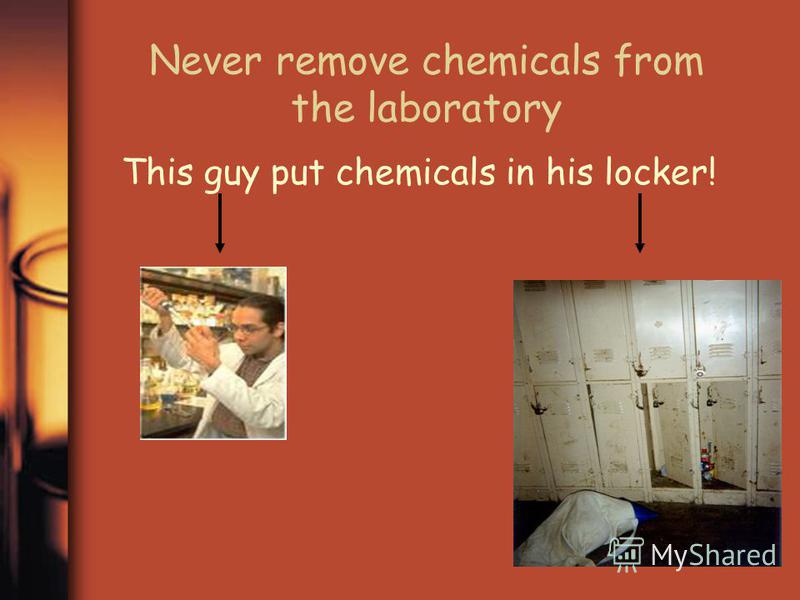The image, resembling a meme or a slide from a PowerPoint presentation, features a brownish-orange background. Dominating the top of the graphic is a cautionary title in light brown text that reads, "Never remove chemicals from the laboratory." Below the warning, another line of text states, "This guy put chemicals in his locker," with an exclamation point. An arrow points downwards from these words to a picture of a young male chemist in a white lab coat, pipetting something into a tube or beaker. Adjacent to this image, another arrow directs attention to a second photo depicting a row of half-sized, dirty, and dingy lockers, some of which are open and possibly contain lab chemicals. The aftermath implies an accident, as the lockers appear damaged. A watermark labeled "my shared" is visible in the lower right corner, and a faintly visible beaker sits partially obscured on the very left side of the background, contributing to the visual context of a laboratory setting.